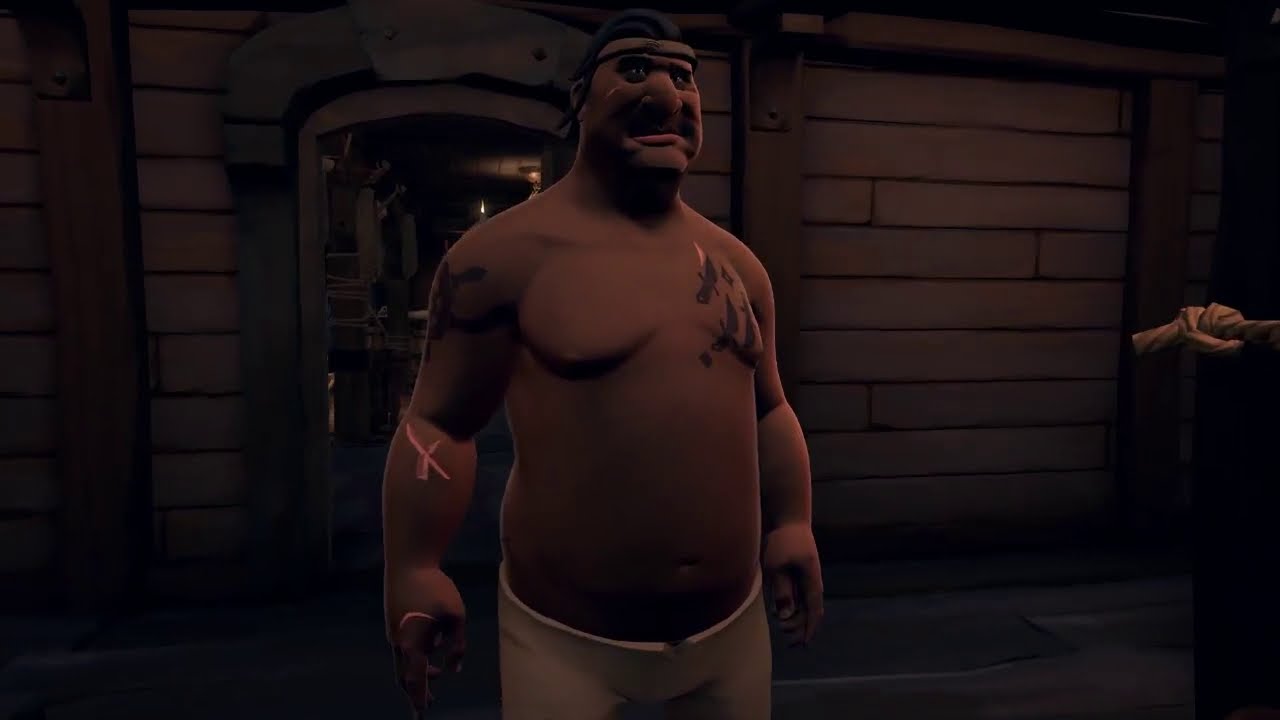The image showcases an animated scene likely from a cartoon, an animated movie, or a video game. Central to the frame is a tall, heavyset man with brown skin, standing topless and exuding an imposing presence. His black hair is complemented by a dark headband, and he sports a black mustache and a notably large nose. His expression is one of anger, emphasizing his intimidating demeanor. He has a very large belly and arms and is dressed in white pants or possibly a white towel tied around his waist. Noteworthy details include a red or pink X-like mark on his right forearm, which might be a scar or a wound, along with tattoos on his right upper arm and the left side of his chest. The background is dimly lit, suggesting an indoor setting faintly illuminated by candlelight. Behind him, the walls appear to be constructed either from long rectangular horizontal bricks or wood boards, adding to the rustic ambiance. Additionally, there seems to be a knotted rope visible on the right-hand side of the image, and faint outlines of hallways and a door frame can also be observed.